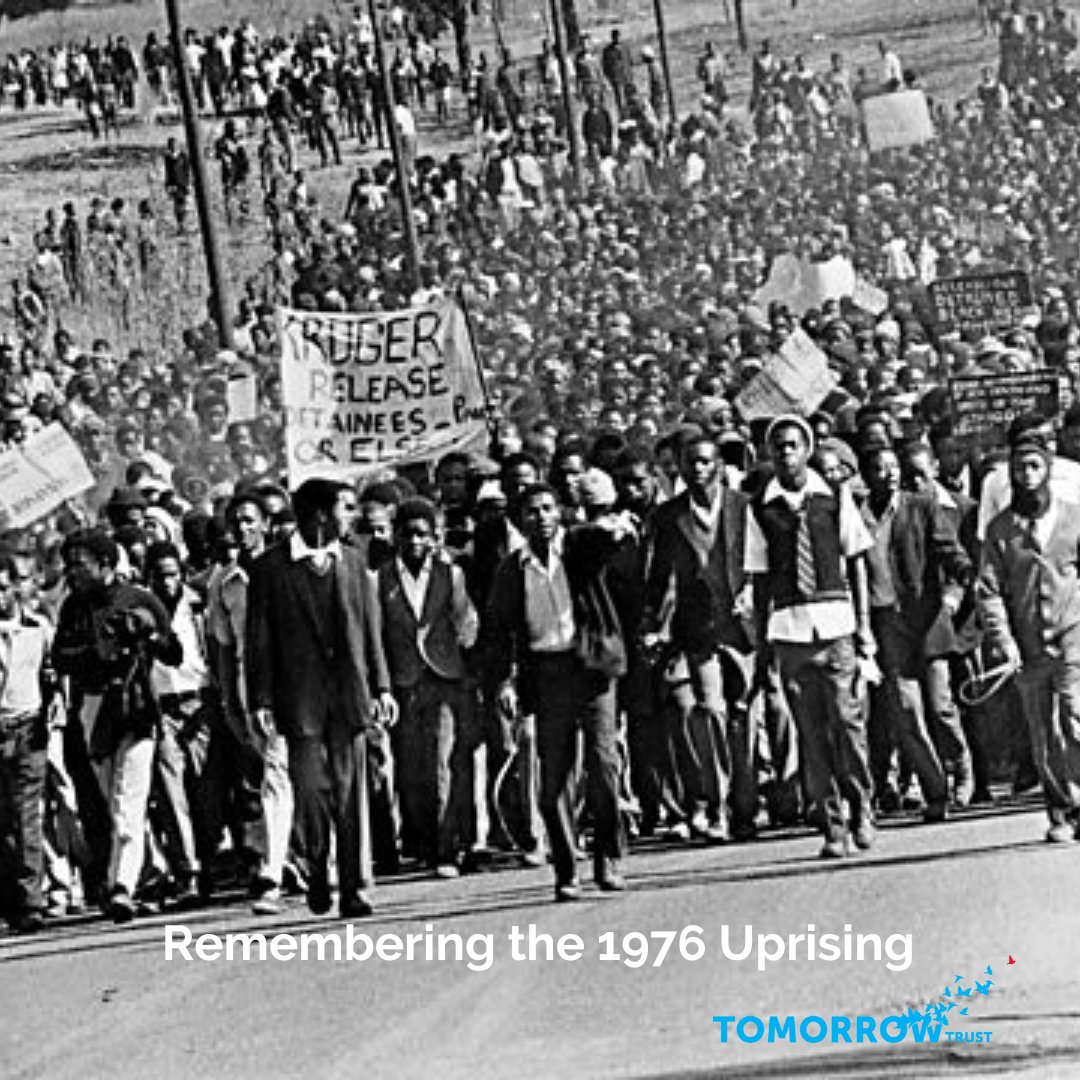This black-and-white photograph depicts a large-scale protest, most likely taking place in the 1970s, as indicated by the associated text at the bottom which reads, "Remembering the 1976 Uprising." The image shows hundreds of predominantly African-American individuals, many of whom are dressed in formal attire, including black pants, black jackets, white button-down shirts, and ties. They are marching down what appears to be an empty highway bordered by grassy fields and a row of telephone poles stretching into the distance. The protesters are holding various signs, with the most prominent one—a white banner—demanding, "Kruger, release detainees or else." The lower right corner of the photograph features the logo and text "Tomorrow Trust" in blue.